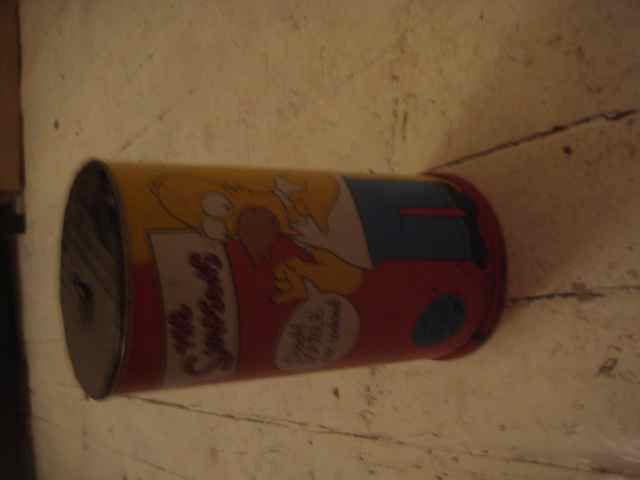A somewhat blurred photograph captures a cylindrical container which could either be made of tin or plastic. The container prominently features a theme from the popular cartoon series "The Simpsons," with the series title displayed on it. The front of the container showcases an image of Homer Simpson dressed in his classic white shirt and blue pants, with his hand raised toward his mouth, apparently eating something or picking his teeth. The container, largely colored in white and yellow, appears to have a black plastic cover similar to those found on Pringles cans, secured with cellophane. There's also a white dialogue bubble next to Homer, although its text remains unreadable due to the image's lack of clarity. The container is placed on a wooden surface, possibly a floor, and the photograph itself is slightly tilted, making it challenging to discern further details.